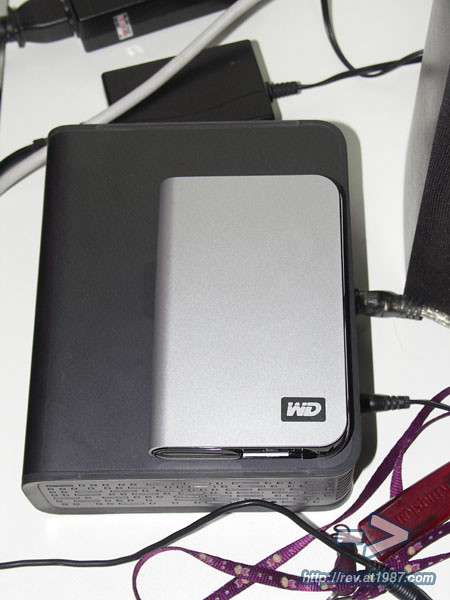The image portrays a cluttered workspace dominated by a black rectangular device, likely an external hard drive or portable battery charger, with a smaller silver box atop it displaying the WD logo, identifying it as a "WD My Passport Elite." This main unit has several cords plugged into it, indicating connections for power and data transfer. The scene is set on a white table, scattered with numerous cables and another black power bank. In the bottom right corner, a purple ribbon or lanyard with a distinctive sideways "V" logo, and the URL http://rev.at1987.com, can be seen, adding to the chaotic yet functional setting.